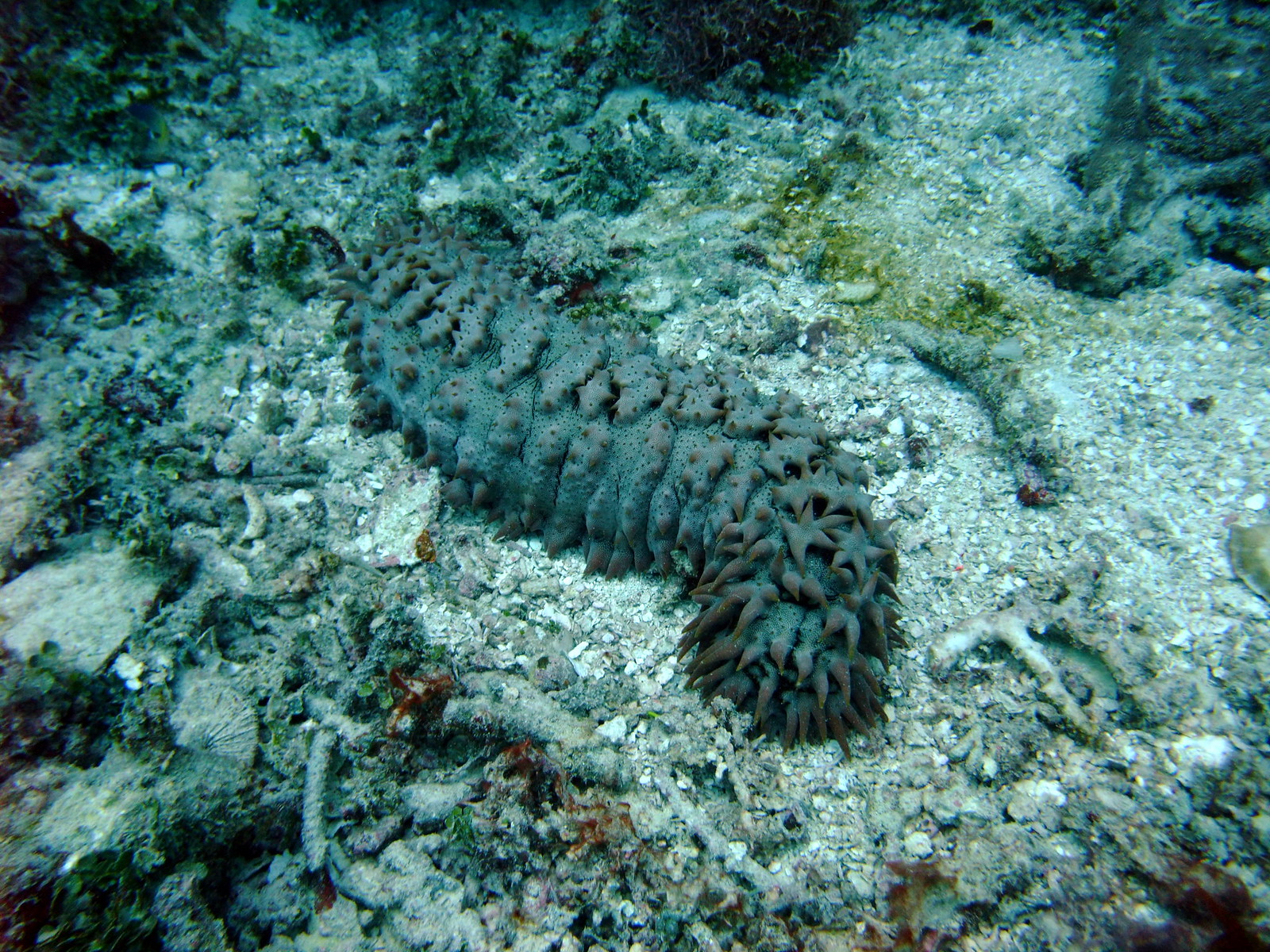This underwater photograph captures the vibrant and diverse ecosystem at the bottom of a body of water. The ocean floor is a grainy, rough surface, scattered with light white and tan rocks interspersed with areas of grayish, lumpy coral. There's abundant marine growth, characterized by green speckles and darker blues that frame the scene.

At the center of the image, a large sea slug takes prominence, appearing gray and segmented. The sea slug features numerous appendages and star-shaped formations, which suggest the presence of starfish or starfish-like structures, blending seamlessly with its body. These appendages have a dark, dingy red hue on their edges, adding to the intricate details of the creature. The sea slug's seemingly symmetrical, five-spoked appendages contribute to its peculiar and somewhat ungainly appearance, adorned with seashells, rocks, and various other marine life. The overall scene is a fascinating glimpse into the complexity and beauty of underwater habitats.